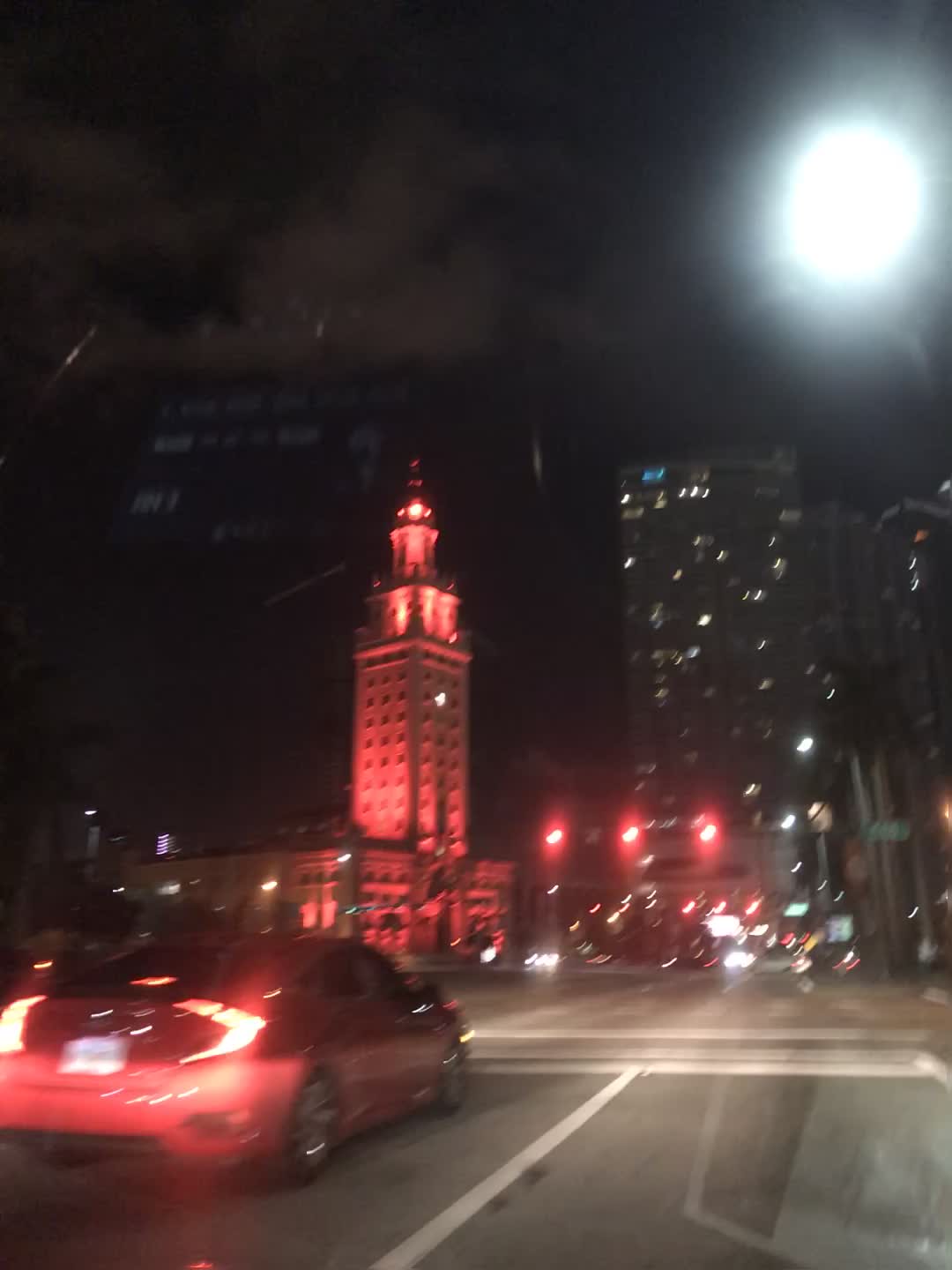This nighttime photograph, taken through a car windshield, captures a vivid city scene. The vehicle is positioned in the right lane of a multi-lane road while a red car is stopped at a traffic light in the adjacent left lane. Ahead, the traffic light displays three glowing red signals, indicating a stop. To the left of the traffic light stands a tall, multi-story building, its façade illuminated in red. In the background to the right, a couple of skyscrapers punctuate the night sky with their sporadic glowing windows. The upper right section of the image features a bright moon surrounded by a halo of reflections. Beneath the traffic lights, a myriad of city lights create a lively urban backdrop. The red car's brake lights are prominently visible, juxtaposed against the white road markings guiding the way ahead.